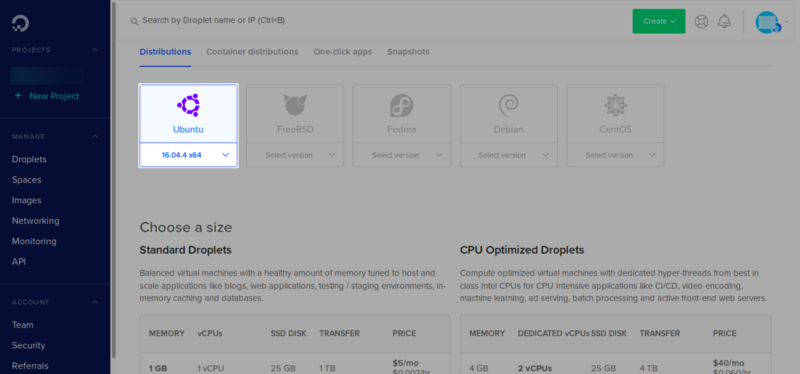This is a detailed screenshot of a web-based dashboard. On the left side, there's a vertical, dark blue navigation panel with a well-organized menu in white font. At the top of this panel, the word "Projects" is prominently displayed. Directly below, there's a white plus sign followed by the label "New Project." Underneath, a series of menu items are listed in a clean, linear arrangement: "Manage," "Droplets," "Spaces," "Images," "Networking," "Monitoring," "API," "Account," "Team," "Security," and "Referrals."

On the right side of the screen, there's a gray background housing the main content area. At the very top of this area is a search field with an accompanying magnifying glass icon and the prompt, "Search by Droplet name or IP (Ctrl + F)." Below this search field is a horizontal menu with categories labeled "Distributions," "Container Distributions," "One-click Apps," and "Snapshots." The "Distributions" tab is currently selected, indicated by its blue color.

In the main section of the content area, five squares are displayed, each containing an icon and a label. From left to right, these squares represent different distributions: "Ubuntu," "FreeBSD," "Fedora," "Debian," and "CentOS." Each icon visually represents its respective distribution, providing a quick reference for users.